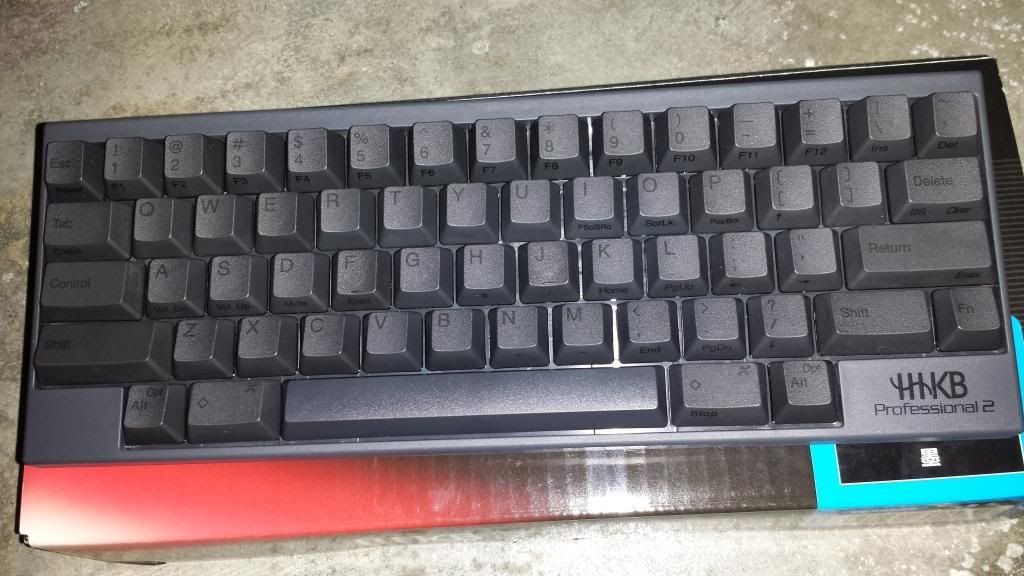The image features a gray external computer keyboard placed against a light brown, mottled surface that resembles a granite countertop. The keyboard and its keys share the same gray hue, with the letters and numbers being a slightly darker gray, making them somewhat challenging to read. Superimposed over the photo is a Photobucket watermark. In the center, "photobucket" is written in very light gray, almost white, lowercase letters. To the left of this text is the Photobucket logo, consisting of circles within circles, creating a three-dimensional effect. Below this, as part of the watermark, is a light gray rectangle with the black text, "protect more of your memories for less!"